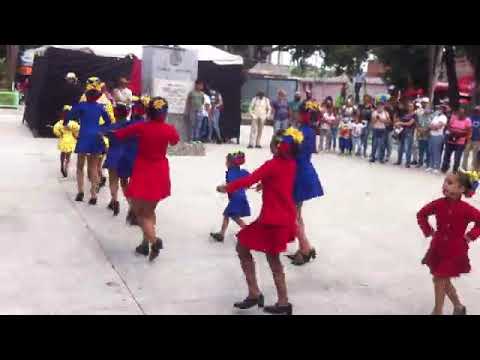This photograph captures a group of young women and girls engaged in a traditional dance or procession in an outdoor setting. They are divided into three groups by color: those at the front wear yellow dresses, the middle group wears blue dresses adorned with red ornaments in their hair, and the rear group is dressed in red dresses with yellow flowers on their heads. All participants wear black high heels, adding uniformity to their appearance. They are marching on a concrete ground, moving towards a black structure with a stone monument at its center. The scene is framed by many onlookers gathered to the right, observing the performers. The background features trees and small buildings, adding depth to the photograph. The image is somewhat low in quality, giving it a pixelated look, and is bordered by two horizontal black strips at the top and bottom.